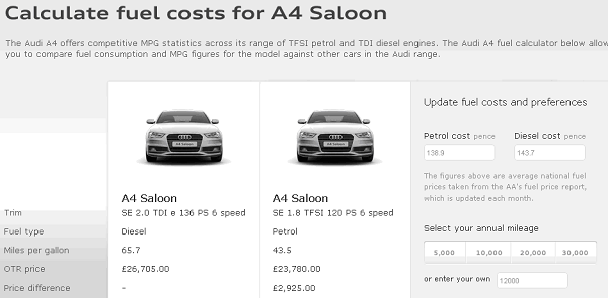Screenshot from a car comparison website with a gray background and black text at the top, reading "Calculate Fuel Cost for the A4 Saloon." Below this header is a brief description, though somewhat obscured, stating that the Audi A4 offers competitive MPG across its range of TFSI petrol and TDI diesel engines. This tool allows users to compare the fuel consumption and MPG figures for the A4 model against other cars in the Audi range.

On the left-hand side near the bottom, there is a table listing the trim, fuel type, miles per gallon (MPG), on-the-road (OTR) price, and price difference for two A4 Saloon models. The first model features an SE 2.0 TDI diesel engine with a fuel efficiency of 65.7 MPG and an OTR price of £26,705. The second model is equipped with a 1.8 TFSI 120 PS petrol engine offering 43.5 MPG at an OTR price of £23,780, thus creating a price difference of £2,925.

Alongside this table, there is an interactive fuel cost calculator allowing users to input the current cost of petrol and diesel, along with their estimated annual mileage. The calculator then computes and displays potential savings or additional costs based on the selected vehicle and entered data.